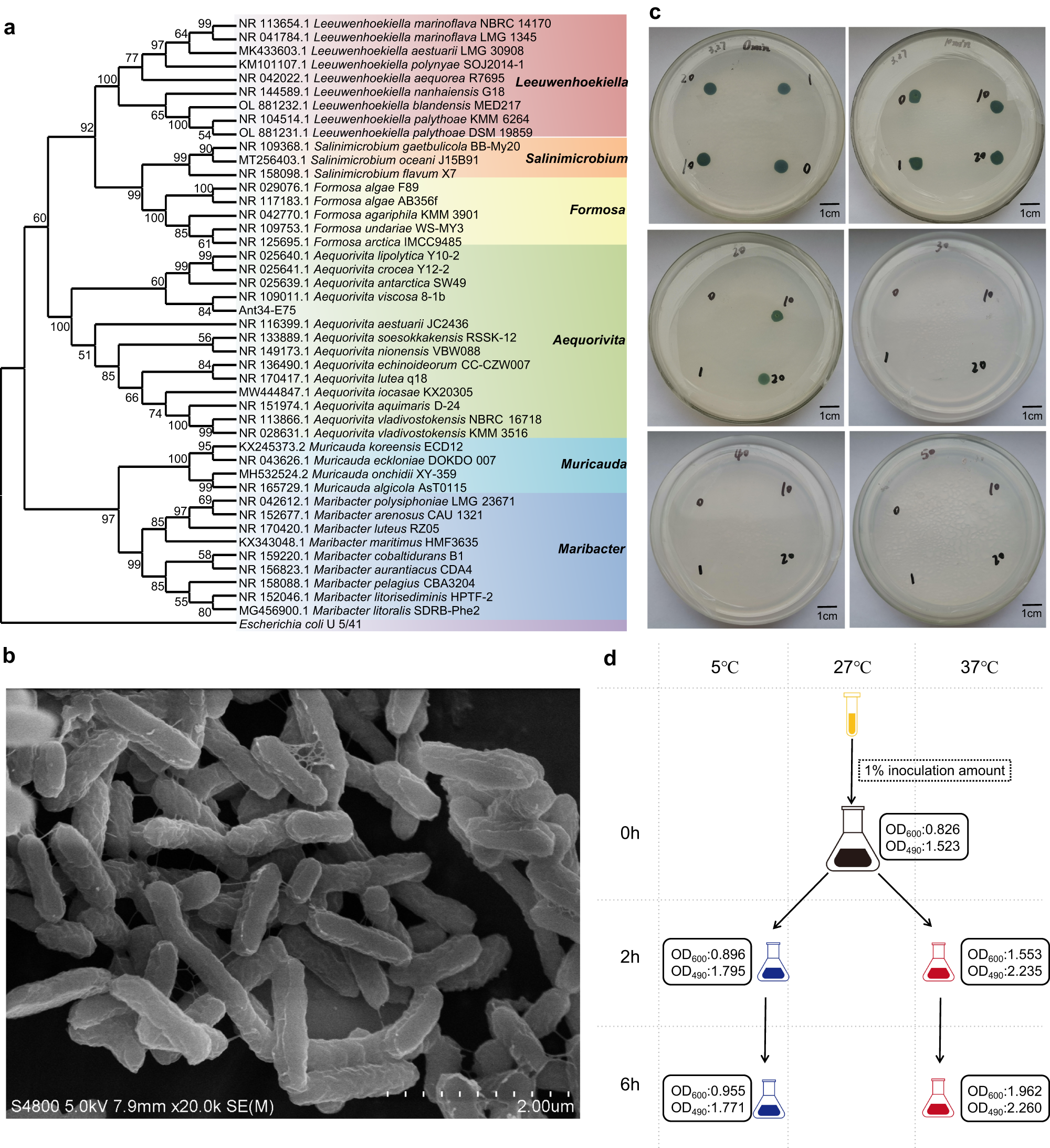This image is composed of four distinct sections, each displaying different types of scientific data, both in graphical and photographic forms. In the top left, labeled as 'A', there's a visually intricate and detailed tree diagram, much like a family tree, that categorizes various entities. This diagram prominently lists names like Luenhochialla, Salinimicrobium, Formosa, Echeverrida, Maricota, and Maribacter. To the right of this diagram, 'B' contains a vertical spectrum of rainbow colors, with red at the top and purple at the bottom, alongside more bacterial names. It also includes a photograph showing light gray, tube-like bacteria against a black background, with annotations such as S4800, 5.0 Kg, 7.9 mm, and magnification details (times 20.0K, SE m). The top right section, labeled 'C’, displays six labeled Petri dishes. These dishes show varying degrees of bacterial growth, with more significant growth in the first three than the last three. In the bottom left, labeled as 'D', there is a detailed microscopic photograph that resembles white, rice-like bacterial structures stacked together. Additional visual elements include a chart with flow arrows connecting beakers, labeled with specific measurements and notations like 1% inoculation amount, evoking a sense of a chemistry lab setting.